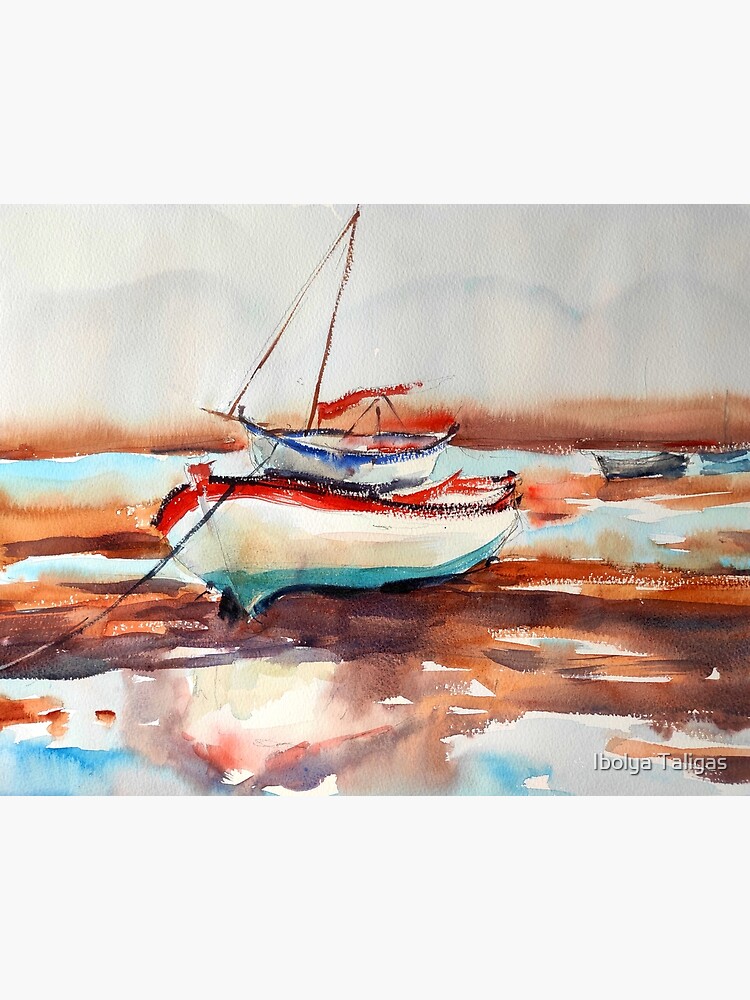This rectangular watercolor painting, approximately 6 inches high and 4 inches wide, depicts a serene maritime scene dominated by two sailboats on a body of hazy, reflective water. The sky occupies the top third of the painting, rendered in a blend of light gray, very pale tan, and hints of light blue, suggesting a cloudy or foggy atmosphere. The water beneath displays an unusual mix of horizontal bands in colors ranging from blue to rust and brown, interspersed with upward brush strokes that give an impression of foliage creeping into the scene.

At the center of the composition floats a small sailboat adorned with red stripes at the top and bottom and white in the middle, complemented by a blue underbelly. A mast rises from its deck, although the sail is currently furled. To the right of this boat, another vessel, painted predominantly in gray, appears almost ghostly, as if it's hovering just above the water's surface. This sailboat lacks a raised sail and is tethered by a rope stretching towards the left side of the frame.

In the lower right corner, a delicate watermark reads "Ebolia Tallegas" in light gray raised print, adding a signature touch to this evocative maritime scene.